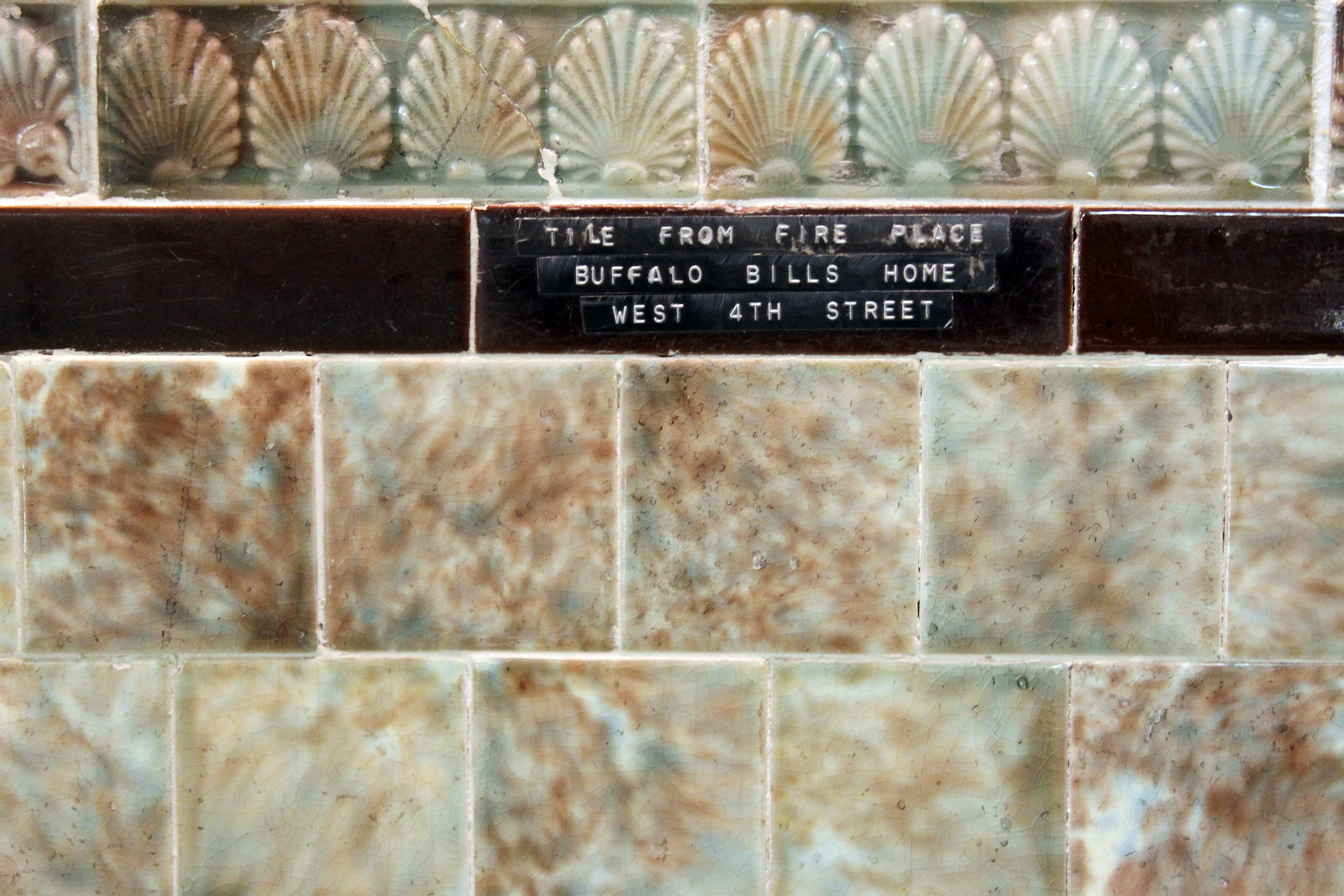This image depicts a horizontally oriented, rectangular section of a tiled wall, featuring three distinct decorative tile sections. At the top, there is a decorative row of rectangular tiles each showcasing an abstract clamshell design with colors ranging from light greenish-blue to red, separated by white grout. Below this, a horizontal layer of dark, either black or brown, subway tiles conceals a message: "Tile from Fireplace, Buffalo Bill's Home, West 4th Street" written in white text. The bottom portion consists of two rows of square tiles featuring a reddish-brown hue with abstract white splotches, separated by white grout, creating a contrast with the darker middle section. This image appears to depict a display wall, showcasing tile specimens that include a historical piece from Buffalo Bill's home.